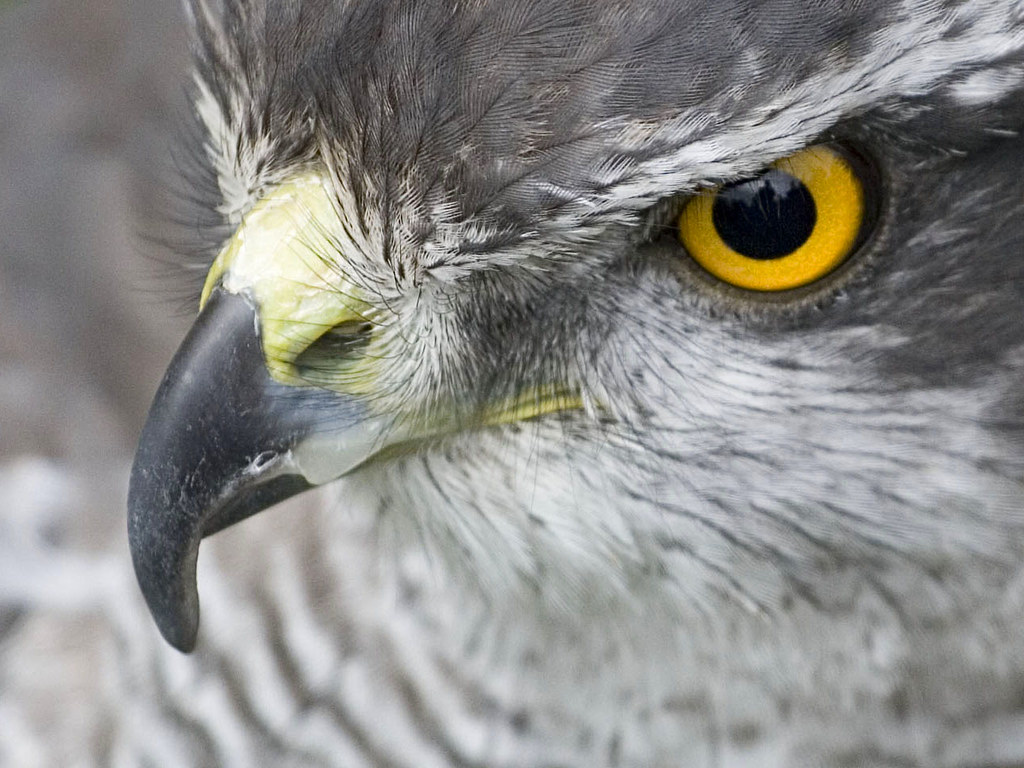This image showcases a magnificent close-up of a bird, likely an owl but possibly a hawk or eagle. The primary focus is on the bird's striking right eye, which features an orange tinge around a deep black pupil, reflecting intricate tree patterns. The bird's head and surrounding area display a mix of dark gray and white feathers, with more white streaks appearing near the eye. Its powerful beak, positioned in the lower left center of the image, is predominantly black with a noticeable yellow protective film at the base. The facial and neck feathers are primarily white with grayish tones, and some black whiskers extend outwards on the left side of its head. The rest of the photo is intentionally blurred, directing full attention to the detailed and vibrant face of the bird.